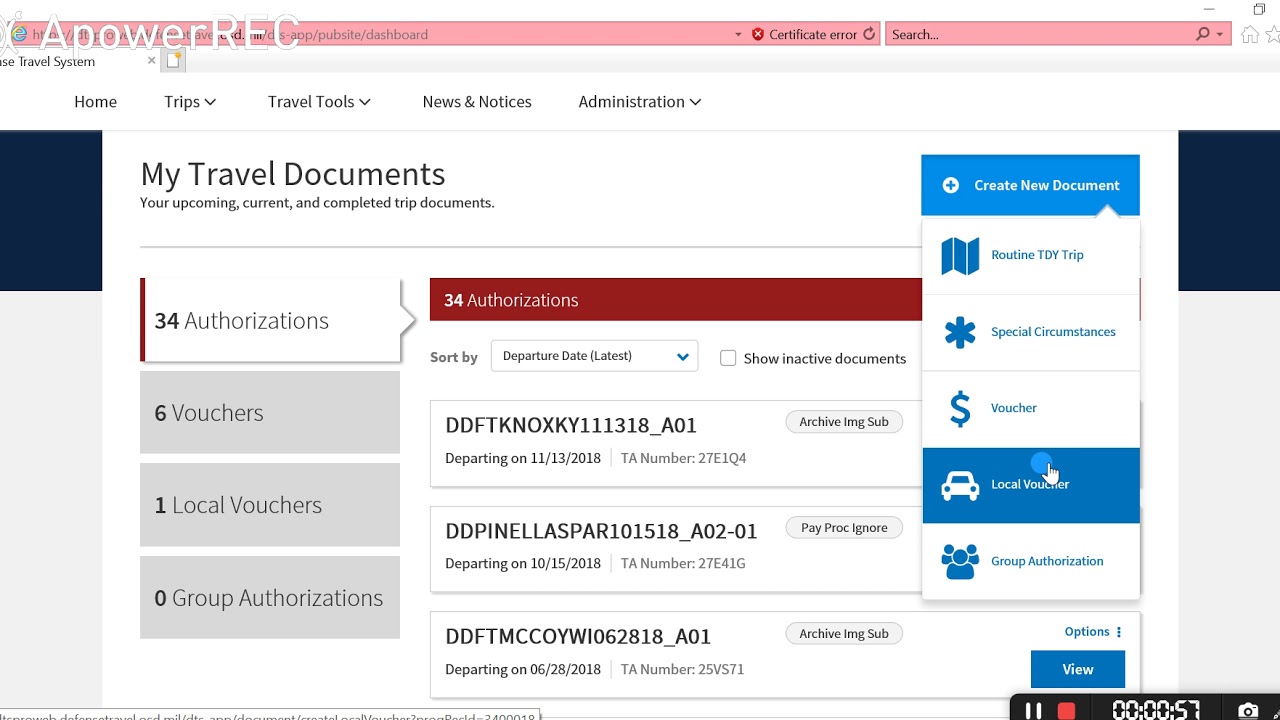This web page belongs to a company named A Power REC, as indicated by the white letters "A Power REC" located in the top left corner of the screen. The top of the webpage features a prominent pink banner that houses the web address, with a matching pink search bar situated on the right-hand side. Below the pink banner is a light gray ribbon, leading into a white background where the main site navigation is displayed in black text: "Home," "Trips," "Travel Tools," "News and Notices," and "Administration." The "Trips," "Travel Tools," and "Administration" options each have a drop-down arrow beside them.

Centrally located on the page, larger black text reads "My Travel Documents," followed by a smaller subtitle in black text stating "Your Upcoming, Current, and Completed Trip Documents." On the far left of the page, there is a vertical ribbon, the top quarter of which is navy blue, with the remaining three-quarters in a pale light blue shade. 

Below "My Travel Documents," there is a vertical drop-down menu on the left side that lists several options: "Authorizations," "Vouchers," "Local Vouchers," and "Group Authorizations." The "Authorizations" option is currently selected. Horizontally across the page is a red banner that reads "34 Authorizations." Beneath this, users have the option to "Sort By" various criteria from a drop-down menu; "Departure Date" is the current selection. To the right of this sorting option is an unchecked checkbox labeled "Show inactive documents."

The main content area features a list of three different documents. Each document is displayed within a horizontal white box, bordered by gray.